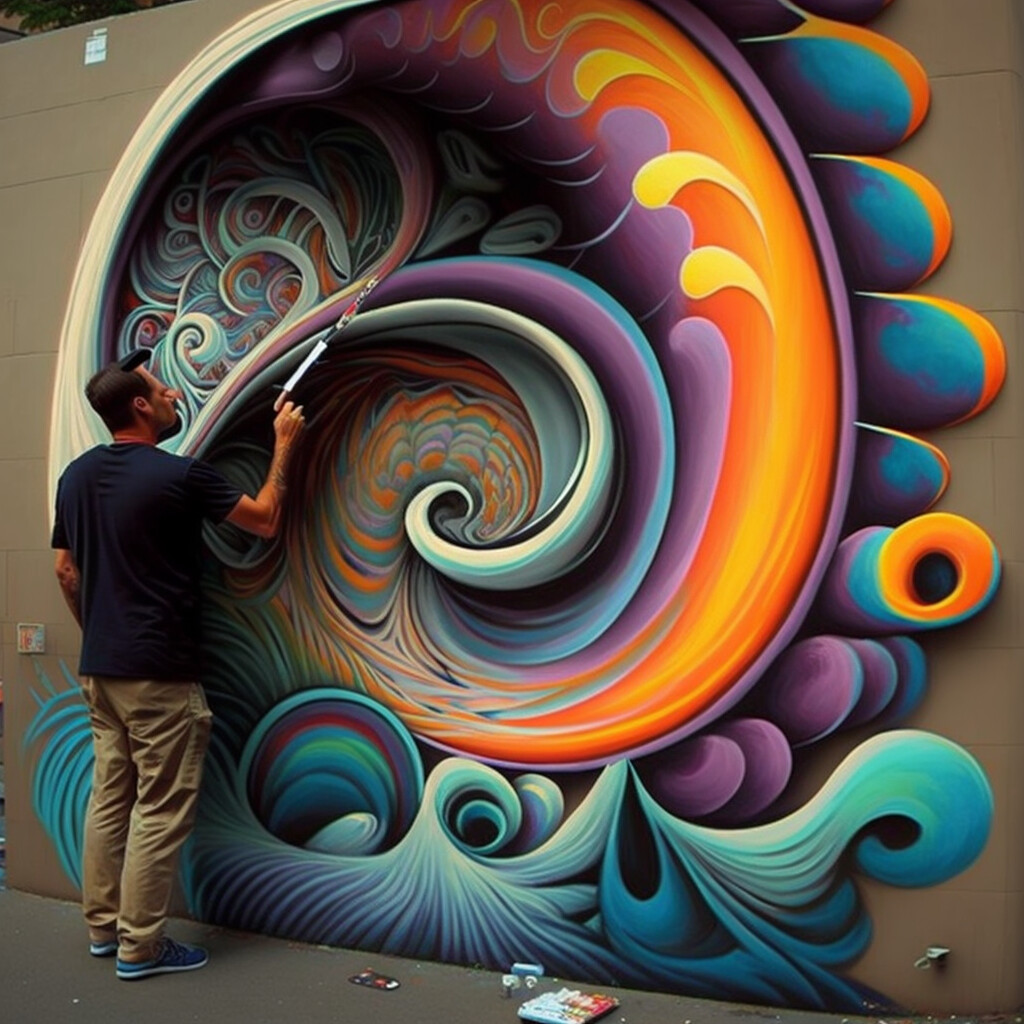This digital painting portrays a man painting a detailed mural on the tan-colored cinder block wall of an outdoor setting bathed in natural light. The man faces away from the viewer, revealing a distorted, cartoonish face. He is attired in a blue shirt, tan pants with large pockets, and blue shoes with white soles. His right arm is bent, holding a silver tube-like paint gun that sprays paint onto the mural. His left arm shows a tattoo, and his brown, short hair partially covers a mustache.

The mural, nearly complete, spans a rectangular area on the wall. It showcases various intricate blue waves at the bottom, symbolizing ocean waves. A prominent feature is a spiral starting with purples and whites in the center, transitioning into blues, purples, and other vibrant colors layered in complex patterns. The outer edges of the mural include textured arcs and layers with shades of yellow, orange, and red, delicately outlined in black, creating a striking three-dimensional appearance. At the top, foliage and part of a building are visible, alongside a small, unclear white sign.

On the smooth, light gray ground beneath the man, various artist supplies are scattered, including a black flat box with colors, a paint palette, and possibly a power outlet. A spigot is visible in the bottom right corner. The intricate mural features additional elements like teardrop shapes, tiny fish, tentacle-like arcing stripes, and more miniature spirals, all contributing to its vibrant and surreal depiction.